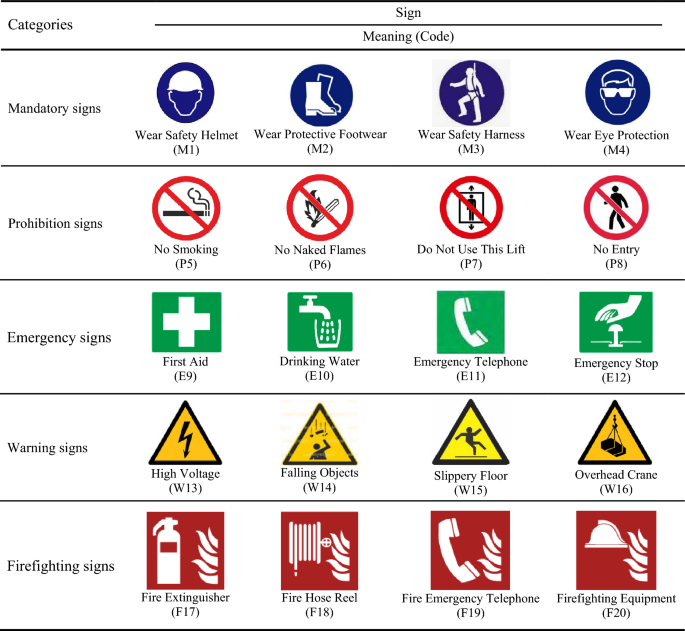A detailed chart designed as a comprehensive legend for workplace signage, typically found in an employee break room, categorizes different types of safety signs using clear icons and color codes. The chart is divided into five main sections:

1. **Mandatory Signs** (depicted in blue): These include directives such as "Wear Safety Helmet" (represented by a figure wearing a helmet), "Wear Protective Footwear" (icon of boots), "Wear Safety Harness" (depicted by a harness icon), and "Wear Eye Protection."

2. **Prohibition Signs** (depicted in red circles with a diagonal line through them): Examples include "No Smoking" (icon of a cigarette with a slash), "No Naked Flames," "Do Not Use," and "No Entry" (a door with a slash).

3. **Emergency Signs** (depicted in green): These include "First Aid," "Drinking Water," "Emergency Telephone" (icon of an emergency phone), and "Emergency Stop."

4. **Warning Signs** (depicted in yellow triangles): Signs include "High Voltage" (lightning bolt icon), "Falling Objects," "Slippery Floor," and "Overhead Hazard."

5. **Firefighting Signs** (depicted in red squares): Examples are "Fire Extinguisher," "Fire Hose," "Emergency Fire Phone" (telephone with a fire icon), and "Firefighting Equipment."

Each category is clearly labeled in black text, with corresponding icons to the right, making it easy for employees to quickly understand and adhere to safety protocols.